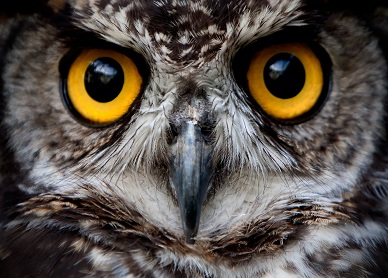This stunning close-up photograph captures the intense gaze of an owl, focusing primarily on its striking eyes and beak. The owl's large, mesmerizing eyes are a brilliant gold with jet-black pupils, with the sunlight reflecting in the irises, making them appear even more vivid. Its sharp, downward-pointed beak stands prominently beneath the eyes. The feathers around the owl's face display a beautiful array of colors, including dark and light browns, whites, and hints of black, forming intricate patterns that surround its eyes and beak. The photograph isolates just the owl's face, excluding its ears and most of its body, highlighting the intensity and detail of its facial features. The background fades into darkness, ensuring all attention is on the striking visage of the owl.